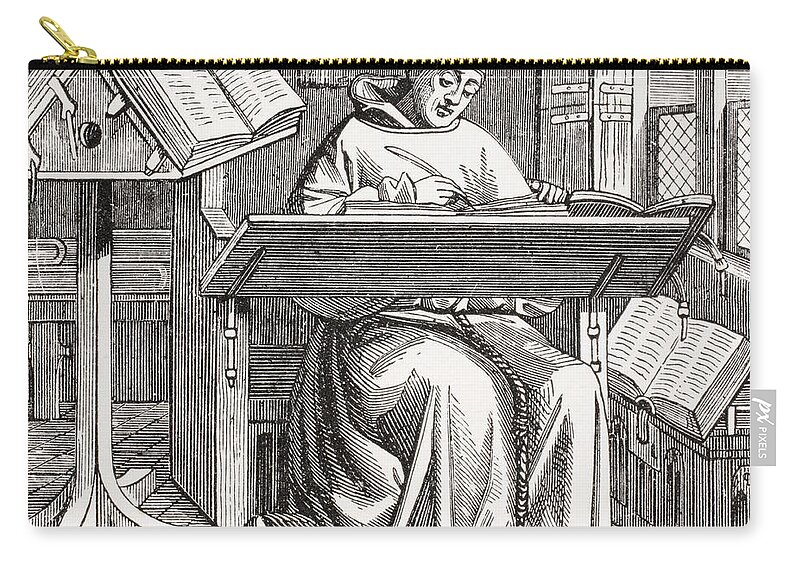This image features a rectangular makeup bag or small pouch with a gold zipper on top and a tag on the right side that reads "PX Pixels." The pouch is adorned with a detailed black-and-white line drawing reminiscent of an old-fashioned style. The artwork depicts a robed monk, identifiable by his rope belt, sitting on a large wooden seat. In front of him is a tilted desk flap holding an open book into which he is writing with a feather quill. To the monk's left is a short table with another open book, its pages filled with lines representing text. Additionally, there is a higher pedestal stand also to the left, closer to the monk's head height, supporting another open book. On the right side, a window is visible, adding to the setting that suggests a scene of diligent study or writing. The top of the monk's head is cut off by the frame's edge.